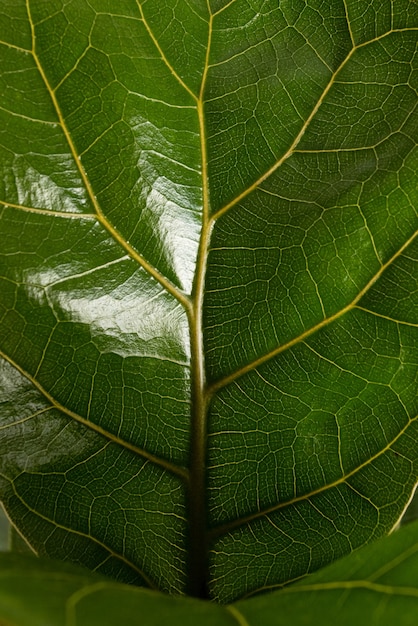This macro photograph showcases a very large, close-up view of a thick, glossy, deep verdant green tropical leaf. The image captures the center of the leaf, dominated by a dark green stem that gradually transitions to a lighter, almost yellowish hue with smaller white and yellow veins radiating outwards. These veins branch alternately from the central stem, resembling a tree trunk with branches extending sideways. The leaf fills the entire frame of the photo, which is displayed in a rectangular vertical orientation. The waxy surface of the leaf reflects highlights from the natural lighting, contributing to the bright and clear setting of the image. The edges of the leaf are not visible, centering the focus on the intricate and highlighted veining pattern. The overall sharpness and clarity of the photograph emphasize the detailed texture and vibrant colors of the leaf.